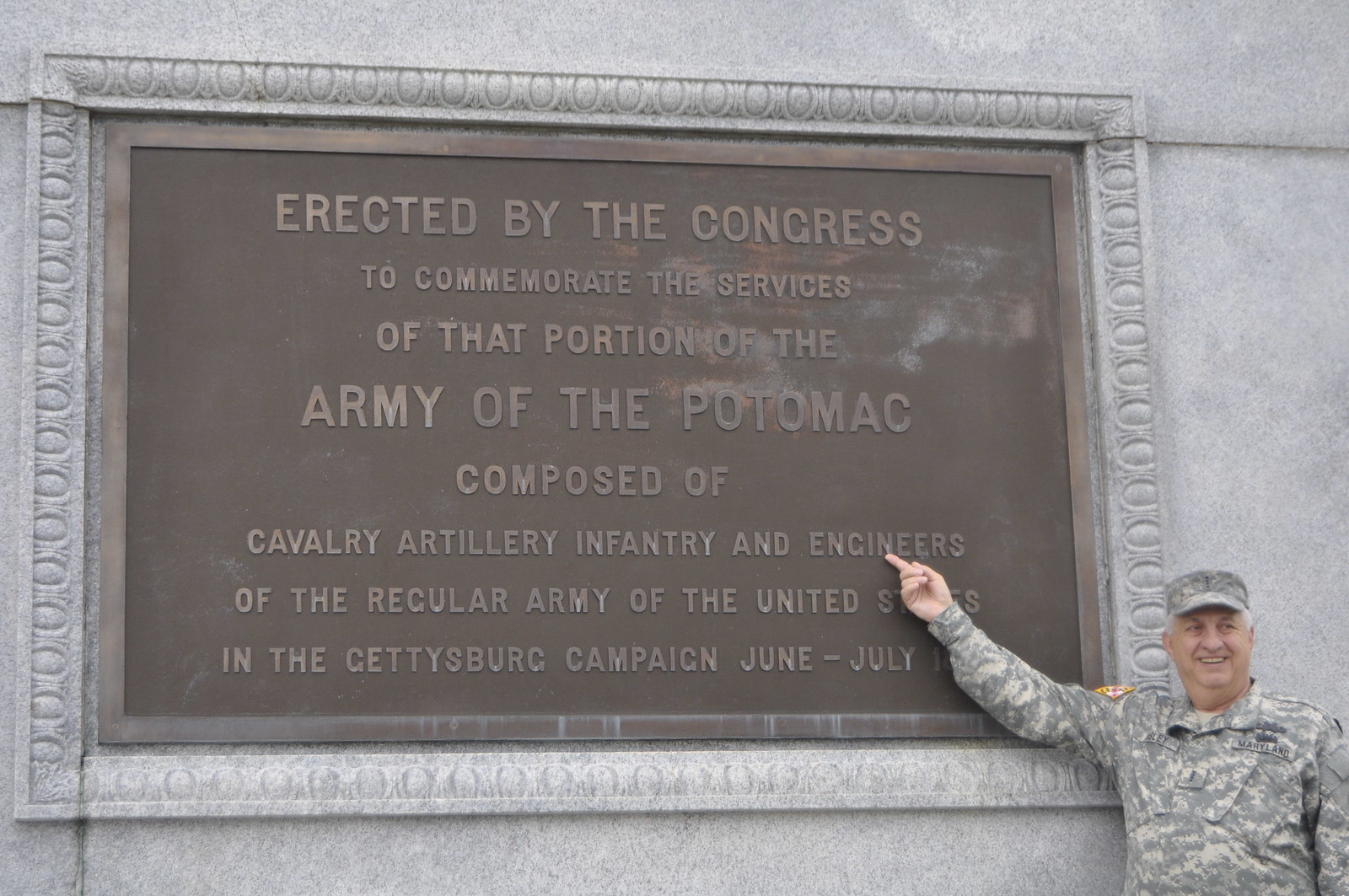In this outdoor image, a soldier clad in military fatigues stands at the lower left corner, pointing with a smile at a large memorial plaque embedded in a towering concrete wall. The plaque, framed by a silver, concrete-like border, is almost as high as the soldier and wider than his height. Made of metal and set against a brown background, the plaque bears an inscription: "Erected by the Congress to commemorate the services of that portion of the Army of the Potomac composed of cavalry, artillery, infantry, and engineers of the regular Army of the United States in the Gettysburg campaign June-July." The soldier’s arm, which is nearly touching the plaque, obscures the precise dates at the end of the inscription. Notable details on his uniform include the Maryland flag on his sleeve and the word "Maryland" on his chest, opposite to where his name is displayed.